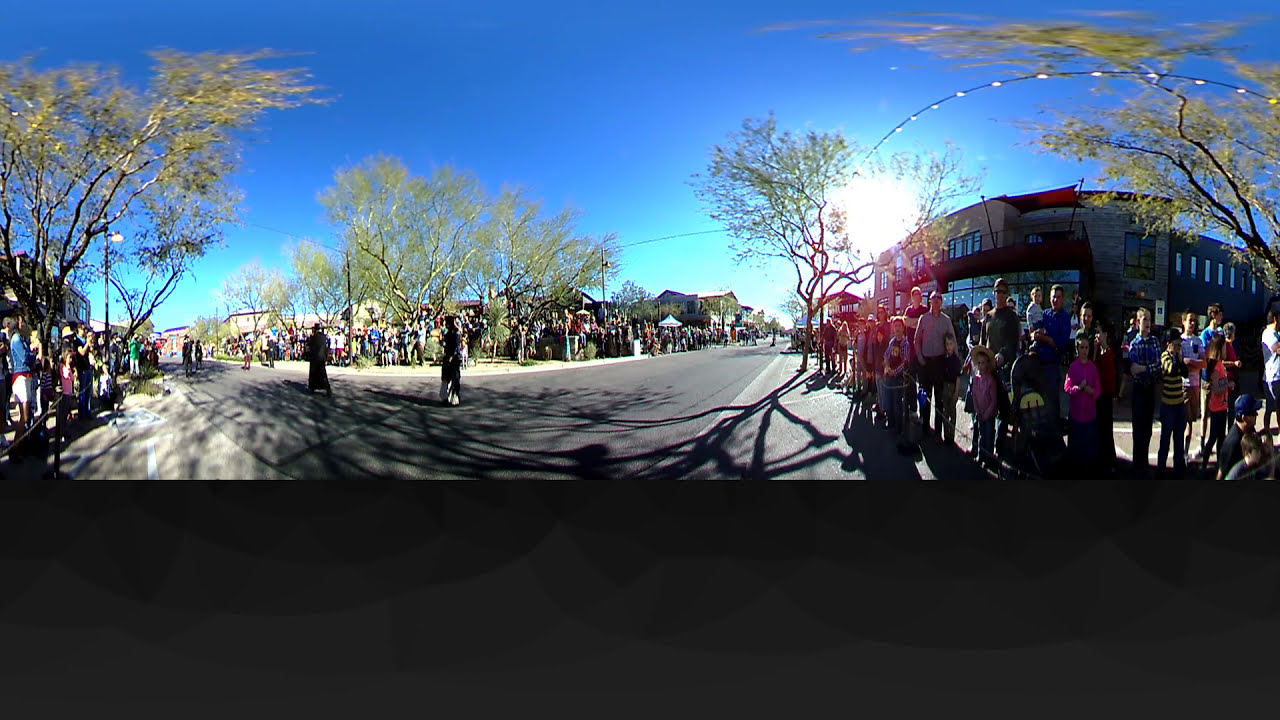The image portrays a bustling, family-friendly public gathering in the middle of a sunny day. Grounded on an asphalt road, the scene is crowded with people lining both sides of the street, which is flanked by a mix of sidewalks and mostly tan buildings with red awnings. The road is clear except for a few individuals walking, predominantly in dark clothing. Many attendees are dressed in an array of colors including blue, pink, and gray. There are a lot of parents with children, suggesting a family-oriented event, possibly a parade. Large trees with green leaves and visible branches dot the background, standing against a clear blue sky. The scene is lively yet scattered, with no single focal point, and no text visible anywhere in the image. A notable feature is a wire strung with lights on the right side, adding to the festive atmosphere.